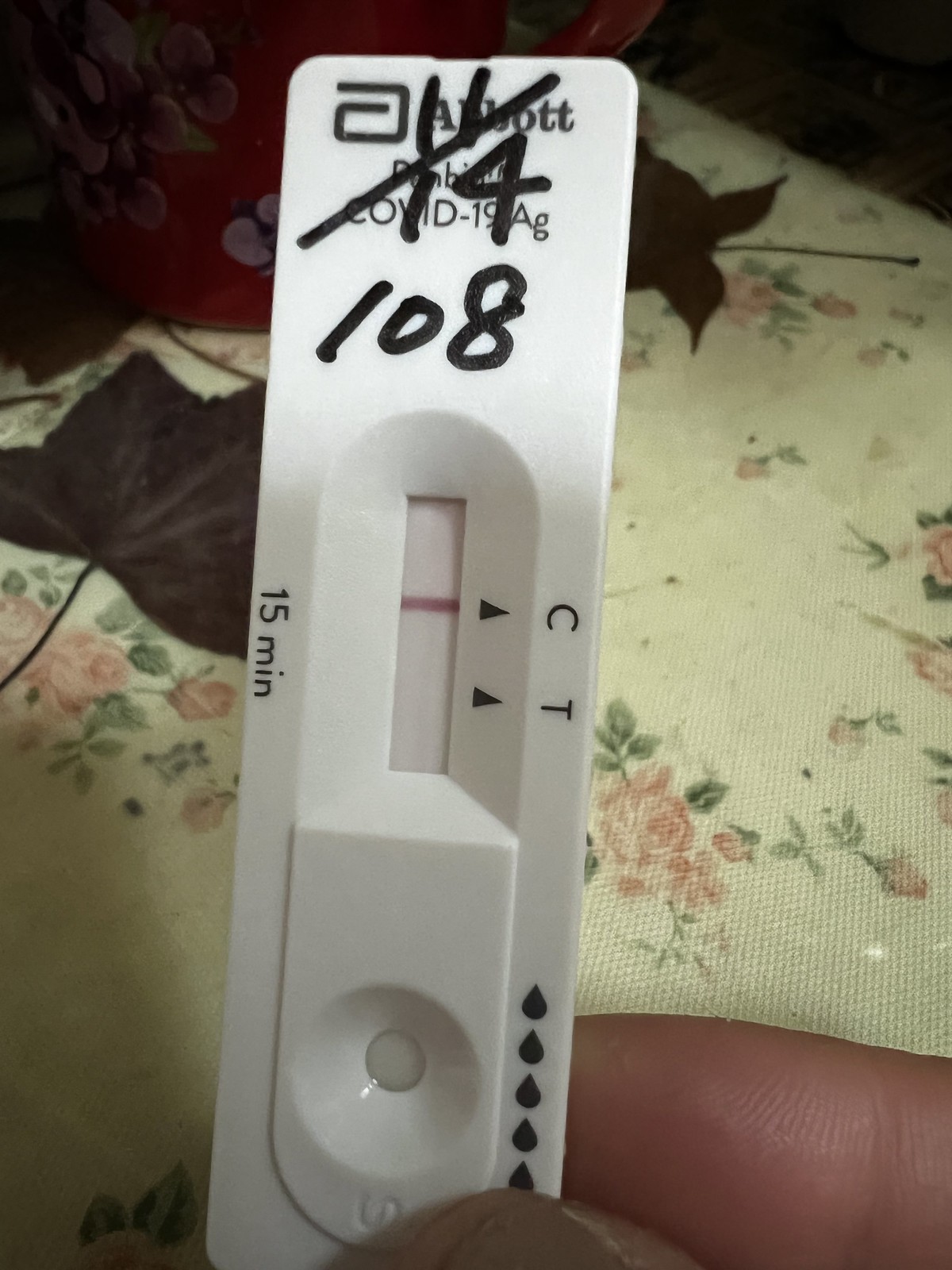The image captures a close-up of a COVID-19 test held by a hand. The test indicates a negative result, with the control line clearly visible and no visible line at the test region. The test device is branded "Abbott," as seen at the top in a professional logo. Above this logo, the fractions "11/14" are handwritten in Sharpie, alongside the number "108."

The backdrop features a white, fabric-like material adorned with a delicate rose pattern, showcasing pinkish roses with green leaves. Adding to the natural theme, two actual green leaves rest on top of the fabric. This intricate background, partially covered by the hand holding the test, provides a soft and aesthetically pleasing contrast to the clinical appearance of the COVID-19 testing device.